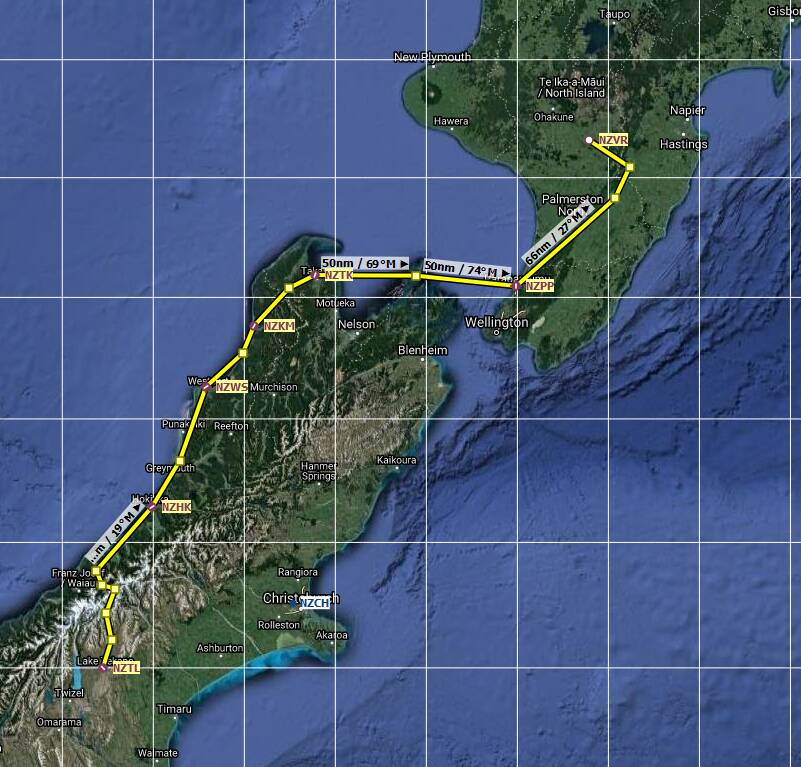The image is a detailed topographic map of New Zealand, featuring a blue background with contour lines indicating ocean depths. Overlaid on this background is a grid of white lines resembling a checkerboard, and additional white lines, possibly added for navigational purposes. The map is likely a zoomed-in view from Google Maps or Google Earth, showcasing both the North and South Islands of New Zealand. Prominent cities such as Wellington, Napier, Hastings, New Plymouth, Christchurch, and others are clearly labeled. There are also various smaller cities such as Taupo, Hawera, Palmerston, Nelson, Blenheim, and many more, including those with Maori names. A bright yellow dotted line, possibly representing a marked route, extends from the southern tip through both islands. Additionally, there are units of degrees of measurement and abbreviations like NZ and VR visible on the map.